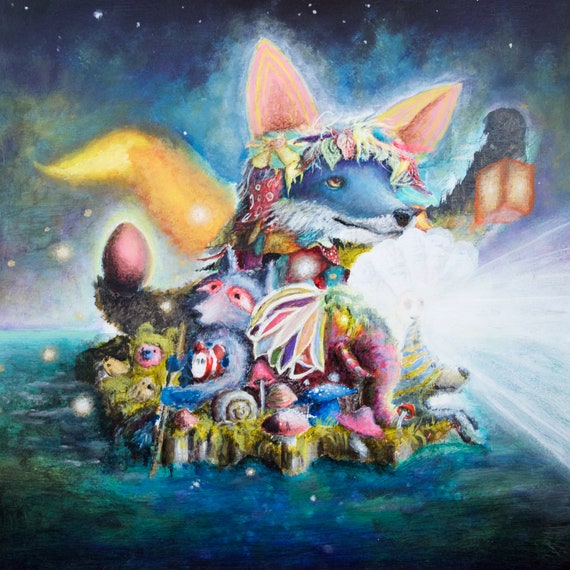The image showcases a vibrant, whimsical scene that appears to be digitally composed or painted, resembling artwork from a children's book. At the center of the image sits a large blue fox with orange and yellow ears, holding up a lantern shaped like a square orange box. The fox, adorned with a rainbow-colored decoration around its head and white fur around its mouth, also has an orange and yellow glowing tail and possibly cradles a pinkish mauve egg in one of its hands. Surrounding the fox on a lush, grass-covered raft or island are various other animals, including a raccoon wielding a paddle and several smaller animals. The scene, set against a backdrop that might be depicting the night sky dotted with stars or galaxies, features colorful toys, mushrooms, and other objects scattered around the island. On the right side, a radiant clamshell emits a bright white light that beams outwards. The greenish-blue water envelops the raft, enhancing the magical and surreal quality of the setting. The island, disproportionately larger than the animals, gives a fantastical feel to the image, blending elements of earth and space.